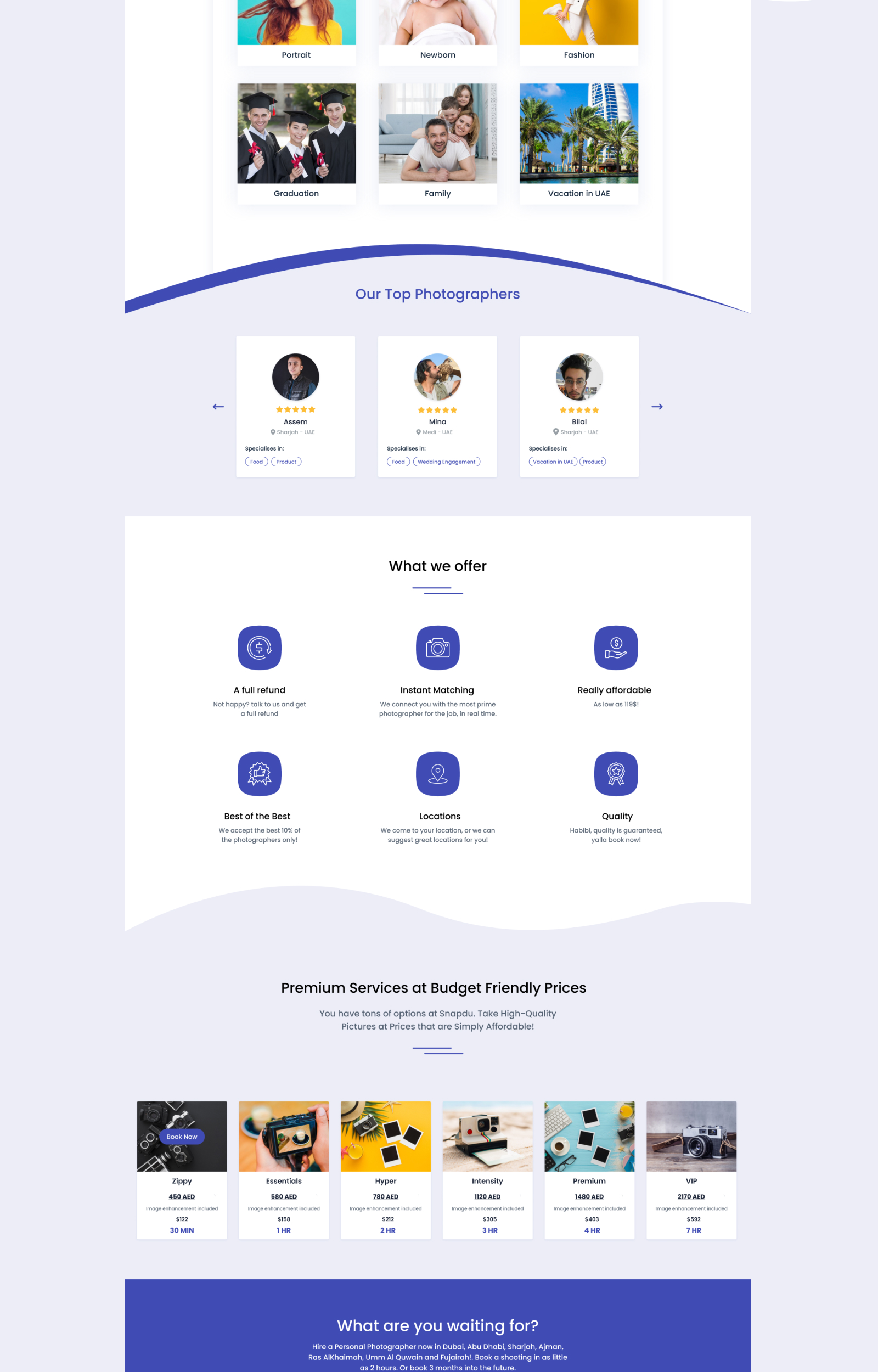This elongated screenshot taken from the Snapdo website showcases their extensive photography services. Despite the small details, the screenshot clearly highlights the top three photographers, all boasting 5-star ratings, with their names and faces displayed prominently. At the top, the navigation menu lists various photography services such as graduation, party events, vacations, weddings, and newborn sessions, although some options are truncated. Below the photographers’ profiles, six informative widgets outline their service guarantees: full refunds for unsatisfactory services, instant matching with photographers, high-quality service, prime locations, and premium offerings at budget-friendly prices. Additionally, Snapdo offers versatile payment options, with prices available in both USD and AED.